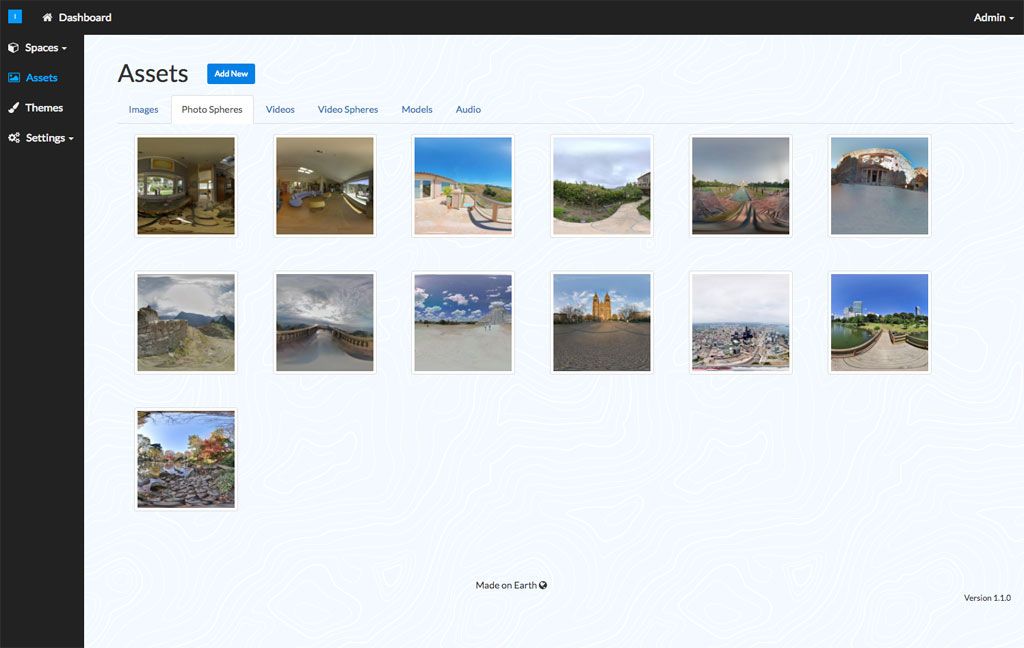The image depicts a web page with a predominantly black background and white details, suggesting a sleek, modern design. At the very top, there's a thin black bar featuring the word "Dashboard" in white text. Down a black column on the left side, you'll find a list of menu items in white, including "Spaces," "Assets" (highlighted in blue to indicate it's selected), "Themes," and "Settings." 

On the right side of this top bar, there's a section labeled "Admin" with a drop-down arrow, implying administrative options. Below, the main content area shifts to a white background where "Assets" is prominently marked in black text, followed by an "Add Image" option in blue.

Further down in this white section, various categories are listed in black text: "Images," "Photos," "Spheres," "Videos," "Video Spheres," "Models," and "Audio." The page showcases 13 thumbnail images arranged in a grid. The first two thumbnails depict indoor scenes, while the third image shows a small pink house set against an outdoor background. The fourth thumbnail features a paved road or walkway bordered by green trees.

The next two images also capture outdoor scenes, and the rest of the thumbnails continue this trend, displaying various outdoor environments. The 13th image appears to be another outdoor scene, completing the diverse collection of visual content.